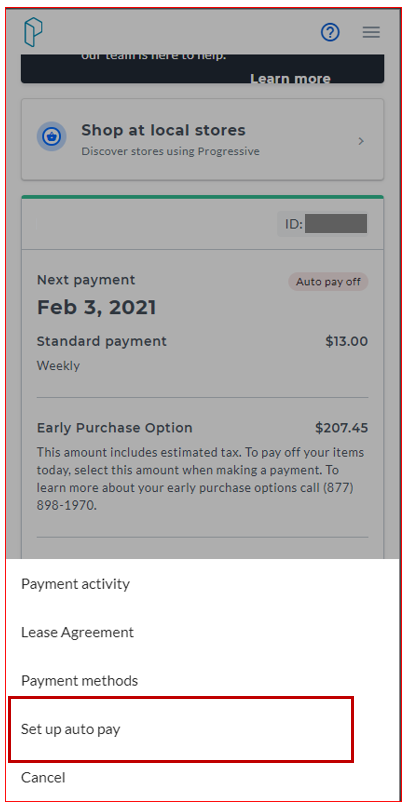This image appears to be a screenshot from an online order interface, designed for interaction with a leasing or payment platform. The background transitions from a light gray at the top to white at the bottom. At the top edge, a black bar contains a "Learn More" link. Below this, a prominent rectangular section displays the text in black letters urging users to "shop at local stores" and to "discover stores using Progressive." 

Following this section, a green line features the label "ID," alongside a gray rectangle awaiting user input for an ID. Below this input field, the next payment date is displayed as "February 3rd, 2021," with an adjacent indicator showing "Auto Pay Off" to the right. 

Descending to the next row, the standard weekly payment is listed as "$13." Below a separating gray line, an "Early Purchase Option" amount is indicated as "$207.45," followed by a detailed description. 

Further down, additional options are presented: "Payment Activity," "Lease Agreement," "Payment Methods," and "Set Up Auto Pay," which is specifically highlighted with a red box. The final option available is the "Cancel" button.